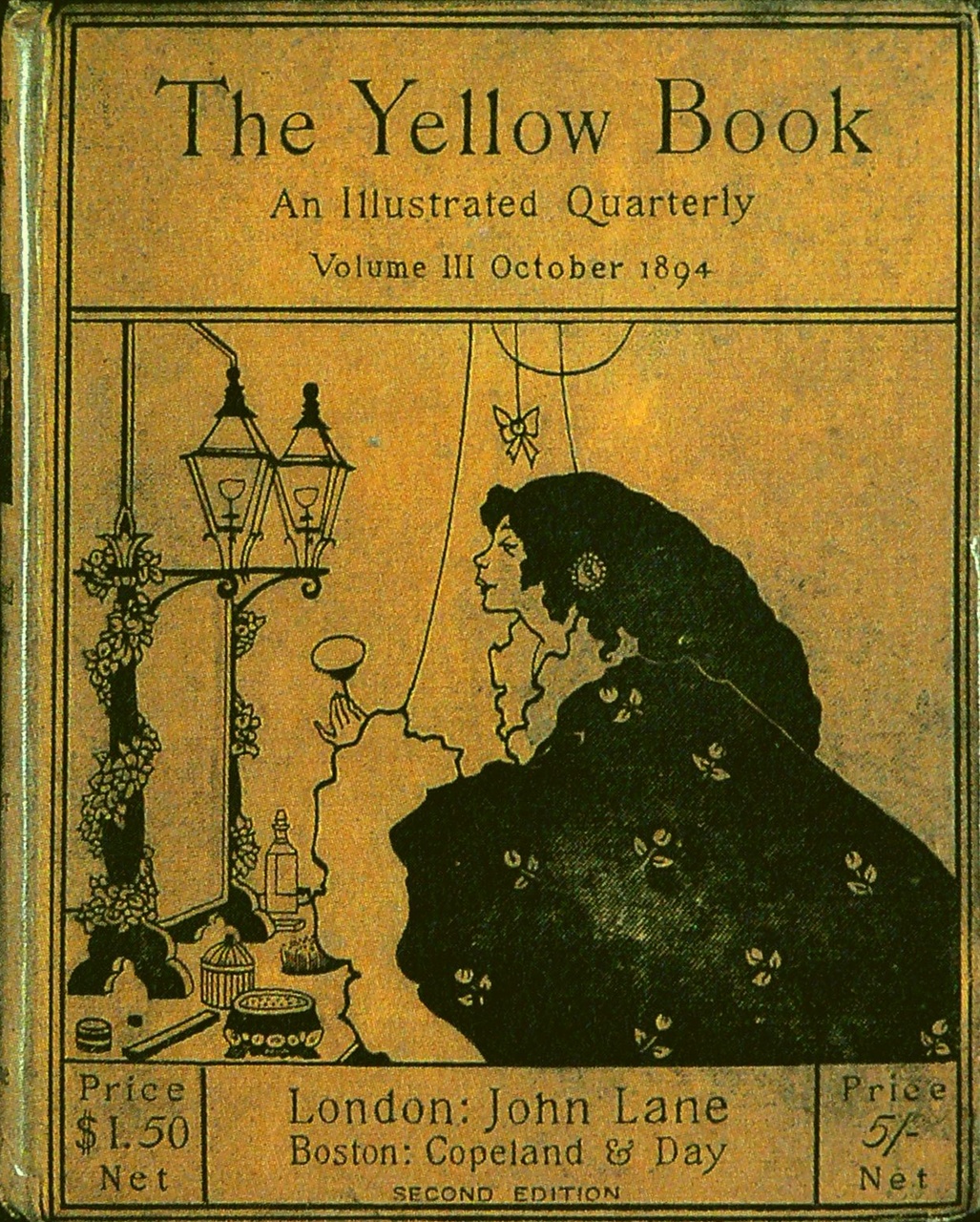This is an image of an old publication known as "The Yellow Book," specifically Volume 3 from October 1894. The cover is yellow with black lettering at the top that reads "The Yellow Book." Beneath this, it is labeled as "An Illustrated Quarterly." Further down, it states "Volume 3, October 1894." Below these details, there is an illustration of a woman with long black hair, dressed in a black gown adorned with floral patterns. She is sitting and facing to the left, appearing to look at a mirror above what could be a makeup table. The mirror, which has distinctive legs on each side, features lantern-like lights at each end. In front of the mirror, various jars and trinkets are displayed. The image also shows a half-circle above the woman's head with strings hanging down, possibly adorned with a butterfly. At the bottom of the cover, additional text reads "Price, $1.50 net" on the left, "London, John Lane" in the center, followed by "Boston, Copeland and Day," and "Second Edition." In the bottom right corner, there is another price indication of "5 cents net." The overall design and details reflect the artistic and historical essence of this late 19th-century publication.